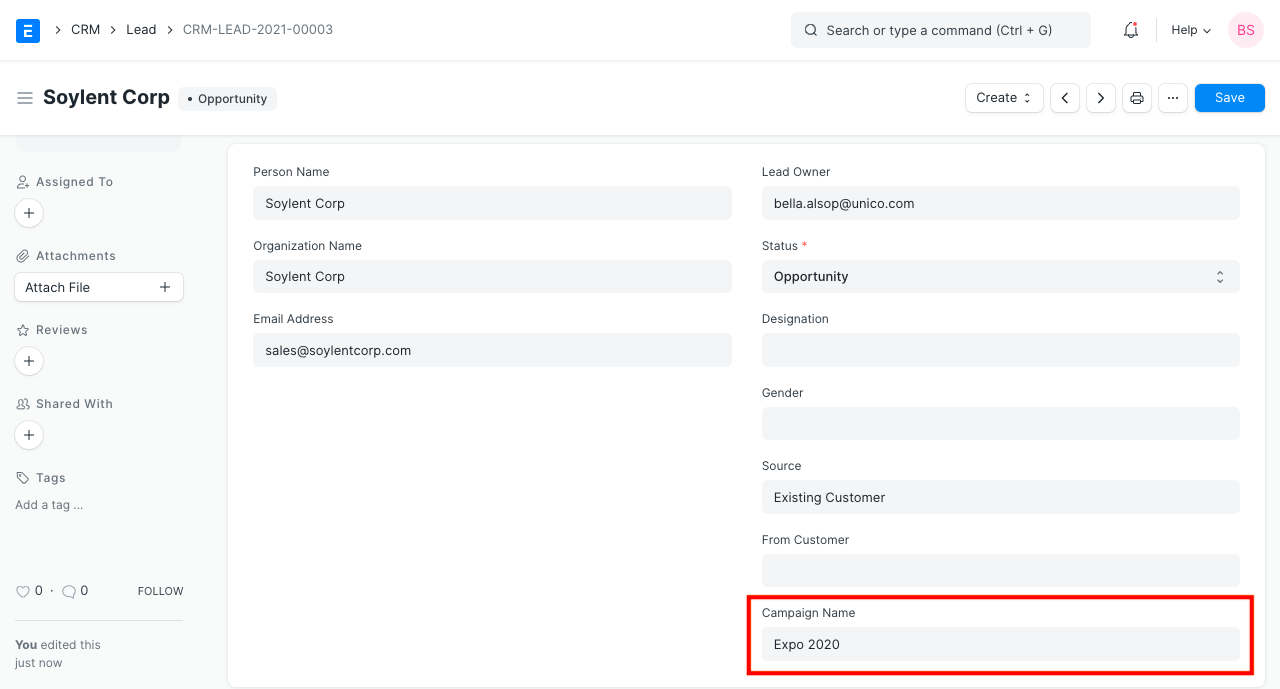**Detailed Caption: Screen Capture of CRM Interface**

The screen capture showcases a section of a CRM (Customer Relationship Management) interface set against a white background with primarily black and gray text. 

**Top Section:**
- A prominent blue box at the top contains a white icon and is labeled "CRM Lead 2021 0000003" in black text.
- Adjacent to this is a gray search box with a magnifying glass icon, stating "Search or type a command, Control + G."
- Nearby, there is a bell icon with a red circle indicator, a help pull-down menu, and a pink circular icon with the letters "BS" in pink.

**Middle Section:**
- Below this line of icons, there are three black lines labeled "Solent Corp."
- A gray box next to it is labeled "Opportunity," followed by multiple other boxes and white pull-down menus.
- Notable elements include a "Create" option, navigation arrows (back and forward), a printer icon, a three-dot menu, and a blue and white "Save" box.

**Left Sidebar:**
- The left section features a vertical arrangement of gray boxes and icons:
  - "Assign To" with a person icon.
  - "Attachments" with a paperclip icon and options to attach files and add new attachments.
  - "Reviews" with a star icon and an option to add new reviews.
  - "Shared With" accompanied by two people icons and a "+” sign.
  - "Tags" with a tag icon and an "Add Tag" option.
- Below these, there are icons for "Heart 0", "Text bubble 0", and "Follow", followed by a timestamp stating "You edited this just now."

**Central Display:**
- The central content area features a white background with various gray boxes, detailing information about "Solent Corp":
  - Person Named: Solent Corp
  - Organization Named: Solent Corp
  - Email Address: sales@solentcorp.com
  - Lead Owner: bella.alsop@unica.com
  - Status: Opportunity
  - Designation: (Blank)
  - Gender: (Blank)
  - Source: Existing Customer
  - From Customer: (Blank)
- A red box highlights the "Campaign Name: Expo 2020."

This organized layout in the CRM interface provides a comprehensive view of the lead and relevant actions.